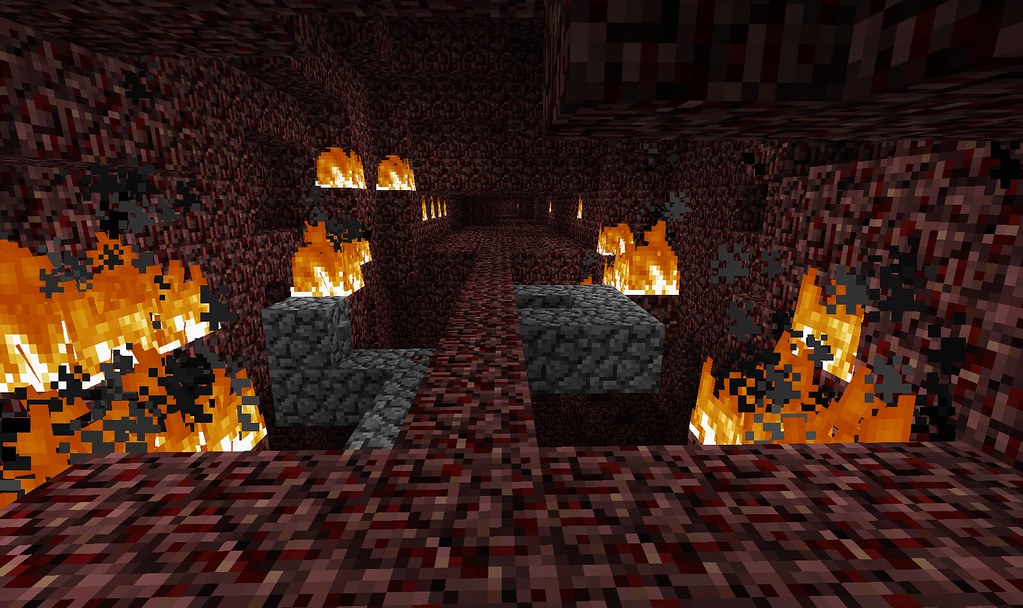This color image appears to be generated by AI or a computer-aided design program, resembling an environment from a video game. The scene is highly stylized and non-photorealistic, characterized by its blocky, geometric aesthetic. The setting seems to depict a cave or cavern, predominantly composed of brown blocks, creating a textured, earthy interior. 

In the center of the image, there is a prominent walkway, also fashioned from the same brown blocks, leading deeper into the cave. Flanking this pathway, on both the right and left sides, are multiple areas depicting fire. These fires are skillfully constructed from square blocks, transitioning from white at the base to yellow and then to orange towards the top, giving it a vibrant, pixelated flame effect.

Additionally, to the sides of the walkway, there are greyish, rocky sections. These areas, made up of roundish but uniformly placed blocks, add a contrasting texture to the scene but maintain the same blocky style, reinforcing the artificial nature of the image. The top of the picture suggests the continuation of the cave into the distance, with darker brown blocks illustrating depth and shadow, leading the viewer's eye further into the cavernous expanse.